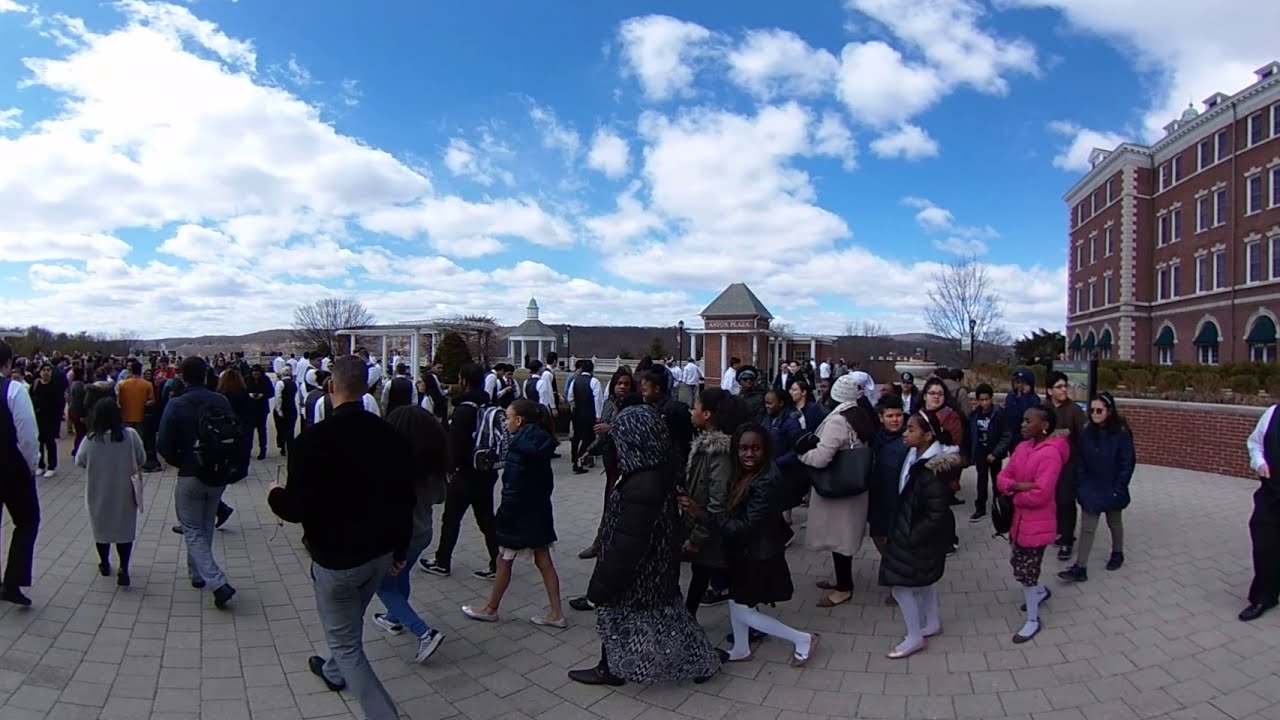A large group of approximately 100 people, including both adults and children, is walking outdoors in a setting resembling a school event or gathering. The crowd, centered in the image, is moving towards the left edge with some individuals branching off to the right. The attendees are dressed in fall or winter attire, with those in the forefront wearing dark-colored jackets, pants, and a notable black teenager in a dark pink sweater. In the background, people in white shirts with black vests and black pants suggest the presence of volunteers or staff in uniform. The scene is set against a cloudy sky filled with cumulus clouds, and the environment features a red brick building with four stories and distinct architectural details, such as arched windows on the ground floor and double sets of purple curtains on the upper floors. The area includes several other structures, a gazebo, and tall rooflines in the distance. The brick walkway and grayish tile grounds enhance the outdoor setting under the cool, blue sky, with deciduous trees missing their leaves emphasizing the fall or winter season.